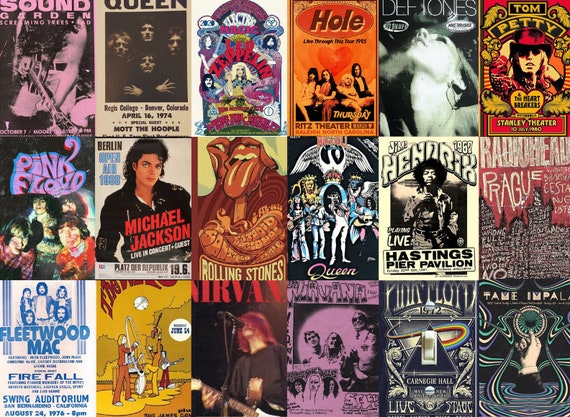The image features a vibrant collage of album covers positioned in three rows, each containing six iconic rock and pop album covers or posters. Showcasing various legendary musicians, the collage includes images of Michael Jackson in his black leather jacket, Queen, Pink Floyd (appearing twice), Led Zeppelin, Hole with an orange background, Deftones, Tom Petty wearing a red hat surrounded by gold, Jimi Hendrix in striking black and white, Nirvana, Fleetwood Mac, Tame Impala, The Rolling Stones with their iconic tongue logo, Soundgarden, and Radiohead. The overall style of the collage is retro, utilizing a wide palette of colors such as orange, red, purple, black, blue, yellow, green, and white, which fills the entire image. Each cover depicts the musicians in varying artistic expressions and positions, making for an intriguing and colorful homage to these influential artists.